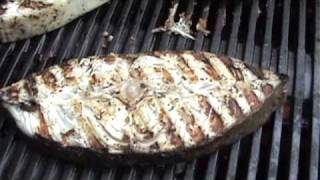The image depicts a close-up view of a couple of oval-shaped pieces of chicken grilling on a black grill with vertical bars. The foreground piece of chicken features distinctive diagonal char marks from the bottom right to the top left, contrasting with its lighter-colored meat. The chicken is white with some brown burn marks and has pointed ends, giving it an almost leaf-like appearance. A smaller fragment of meat is visible, stuck slightly above the main piece, while another similar piece is partially cut off in the top left corner of the image. The black grill has grooves separating its vertical bars, with one long horizontal metal piece running across. The picture is well-lit but of low resolution, showing no other elements like people or utensils, just the grilling chicken.